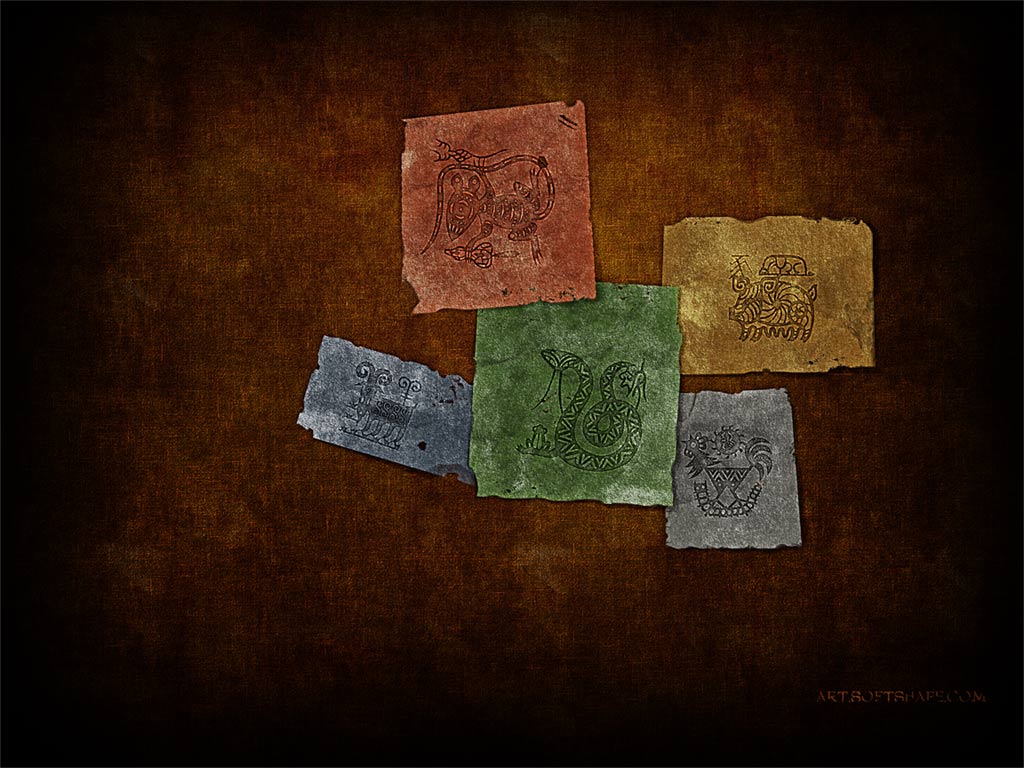This color photograph depicts a dark brown surface, akin to a sponge-painted wall combining hues of red, brown, and gold. Arranged on this surface are five distinct pieces of colored, handmade-looking paper, each varying in size and shape, with a torn quality to their edges. The papers overlap slightly, creating a layered effect: a blue paper on the left, tucked slightly under a green piece, which in turn partially covers a red paper. Beneath the green paper are a yellow piece and a gray piece. Each paper features intricately detailed animal sketches. The green paper showcases a snake with its tail curled and an extended tongue, positioned above a frog. To its left is a blue paper depicting a goat, and above the green paper is another drawing resembling a mouse with a long tail, holding something in its hand. The yellow paper contains an image of a pig, while the grayish-blue paper features a face-like image decorated with patterns of a sun and a bird. Each drawing, whimsical and detailed, lends a unique character to the collage.